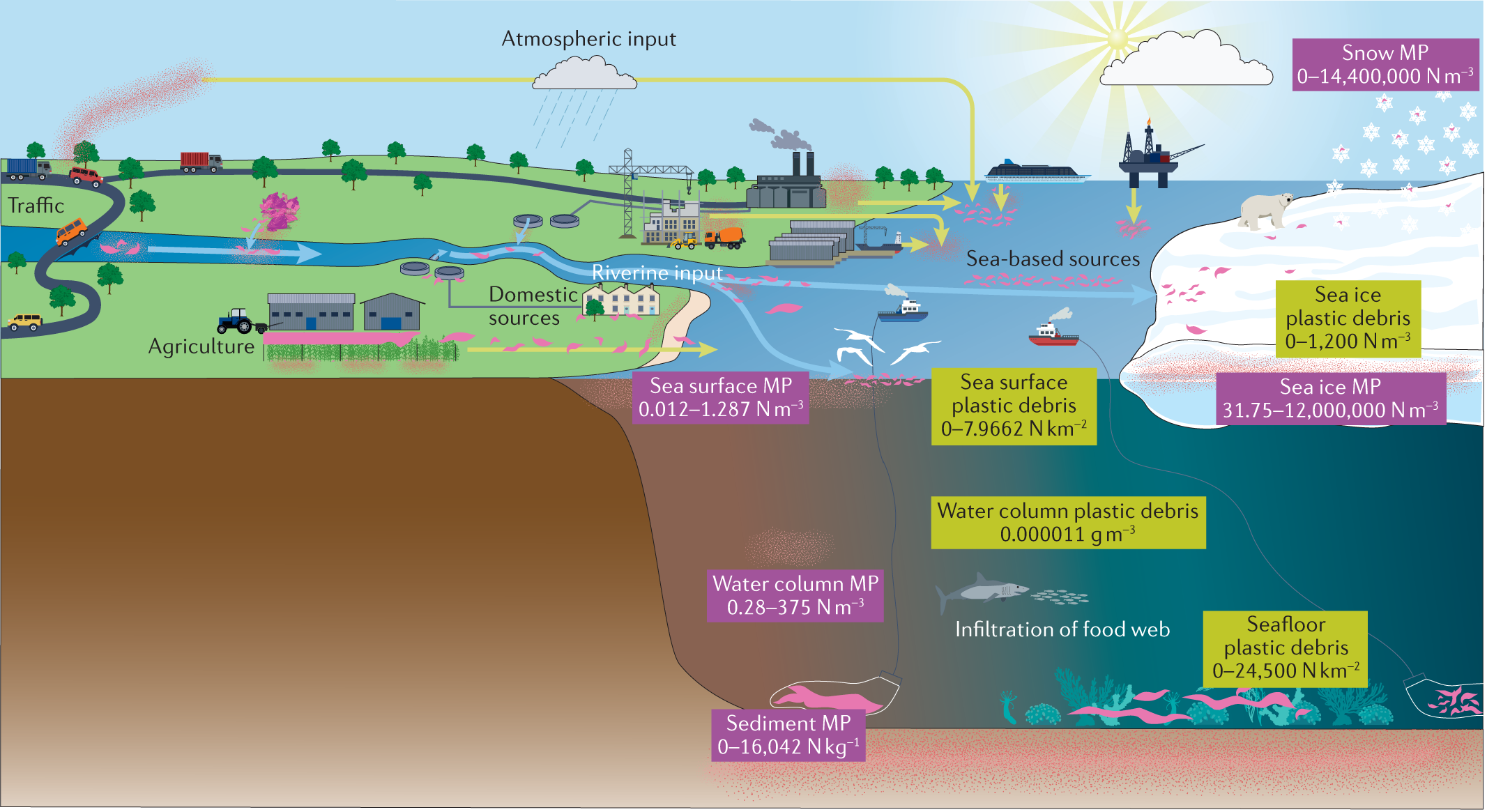The image is a detailed cartoon-style illustration depicting how pollution and plastic enter waterways through multiple sources. On the left-hand side, various land-based sources contribute to the pollution: traffic on roads, agricultural farms with harvested crops, residential areas labeled as "domestic sources," and factories emitting pollutants. This side of the image includes atmospheric input, shown by a cloud, with pollutants being carried by rain into rivers. These rivers traverse the landscape and eventually feed into the ocean. 

In the middle to the right side, the progression of pollution into the marine environment is emphasized. The ocean section displays the plastic debris distributed across different water layers: floating on the surface, suspended within the water column, and settled on the seafloor. Marine life, including fish, is depicted ingesting the plastic, illustrating its integration into the food web.

Additional contributors to marine pollution include sea-based sources. Boats and oil rigs are depicted discharging plastic waste, which is visualized as pink debris through directional arrows. An iceberg with a polar bear sitting atop it highlights the penetration of plastic into ice and snow, emphasizing the far-reaching effects of pollution. The extensive use of textual labels and schematic arrows effectively illustrates the various pathways through which plastic pollution spreads from land and air into marine environments, affecting ecosystems at multiple levels.